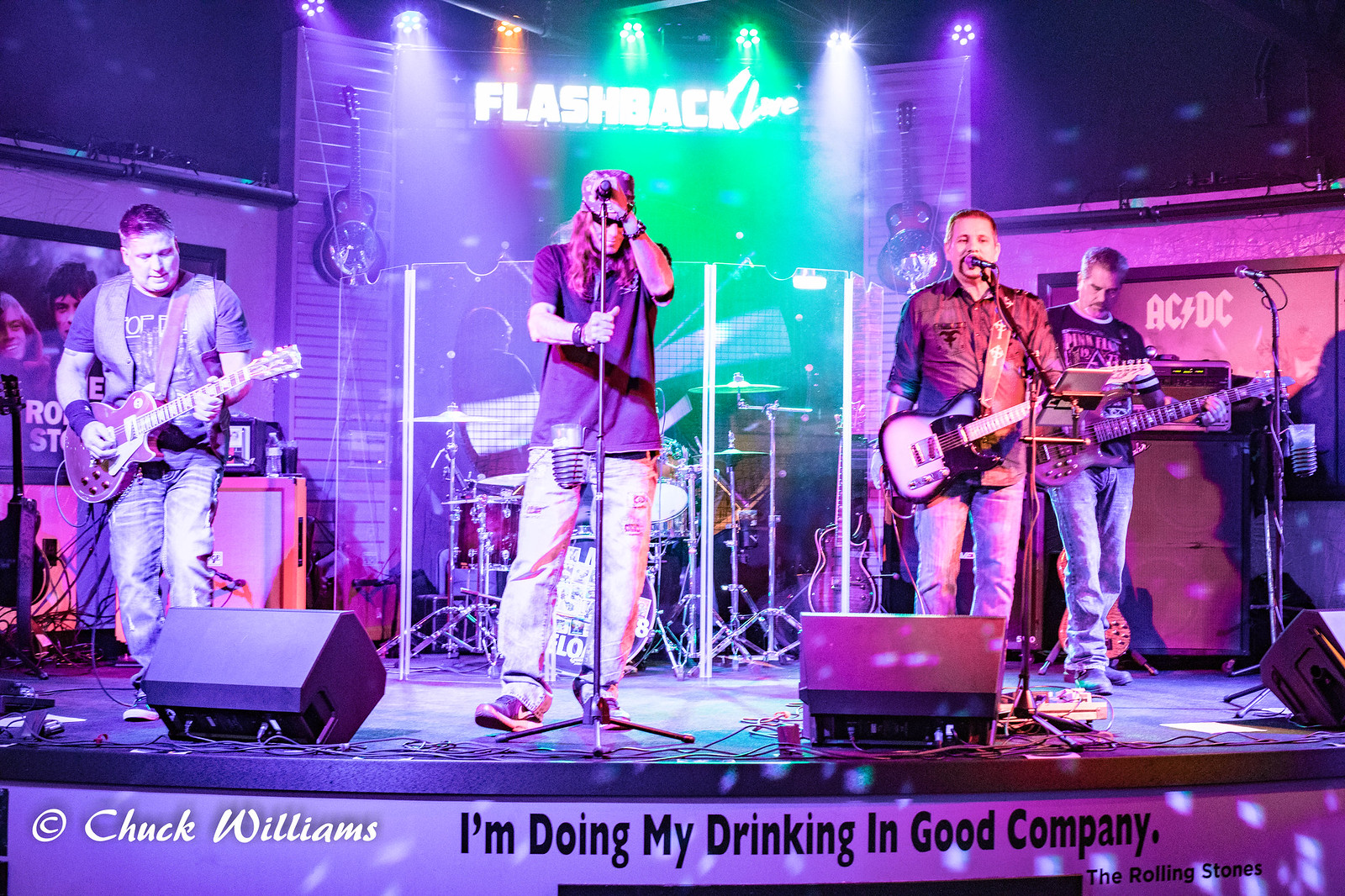This is a horizontal rectangular photograph capturing a live band performance in what appears to be an indoor stadium or concert hall. The stage is bathed in vibrant purple lights, punctuated by flashes of green and orange from the light bars above, transitioning from purple on the left, to orange and green in the middle, and back to purple on the right. The background of the stage remains dark, rendering some elements indistinguishable.

Prominently displayed across the backdrop is the partial word "flashback," hinting at a nostalgic theme, with another unreadable word beside it. Center stage stands the lead singer, a Caucasian man donning a bandana, gripping a microphone stand and the microphone itself with a commanding presence. Flanking him on both sides are guitarists: to the left, a Caucasian man playing an electric guitar, and to the right, another guitarist closely situated near a microphone, apparently taking the role of a co-vocalist but not currently playing his guitar. Behind these musicians looms a drum set, with the faint silhouette of the drummer just visible.

Adding to the ambiance, the wall at the back of the stage features a sign that says "ACDC," and a Rolling Stones picture is discernible on the far left-hand side. At the front bottom left of the stage, there's a white-printed copyright mark reading "© Chuck Williams." In the center bottom area, black text declares, "I'm doing my drinking in good company the Rolling Stones," adding a touch of rock 'n' roll ethos to the scene.